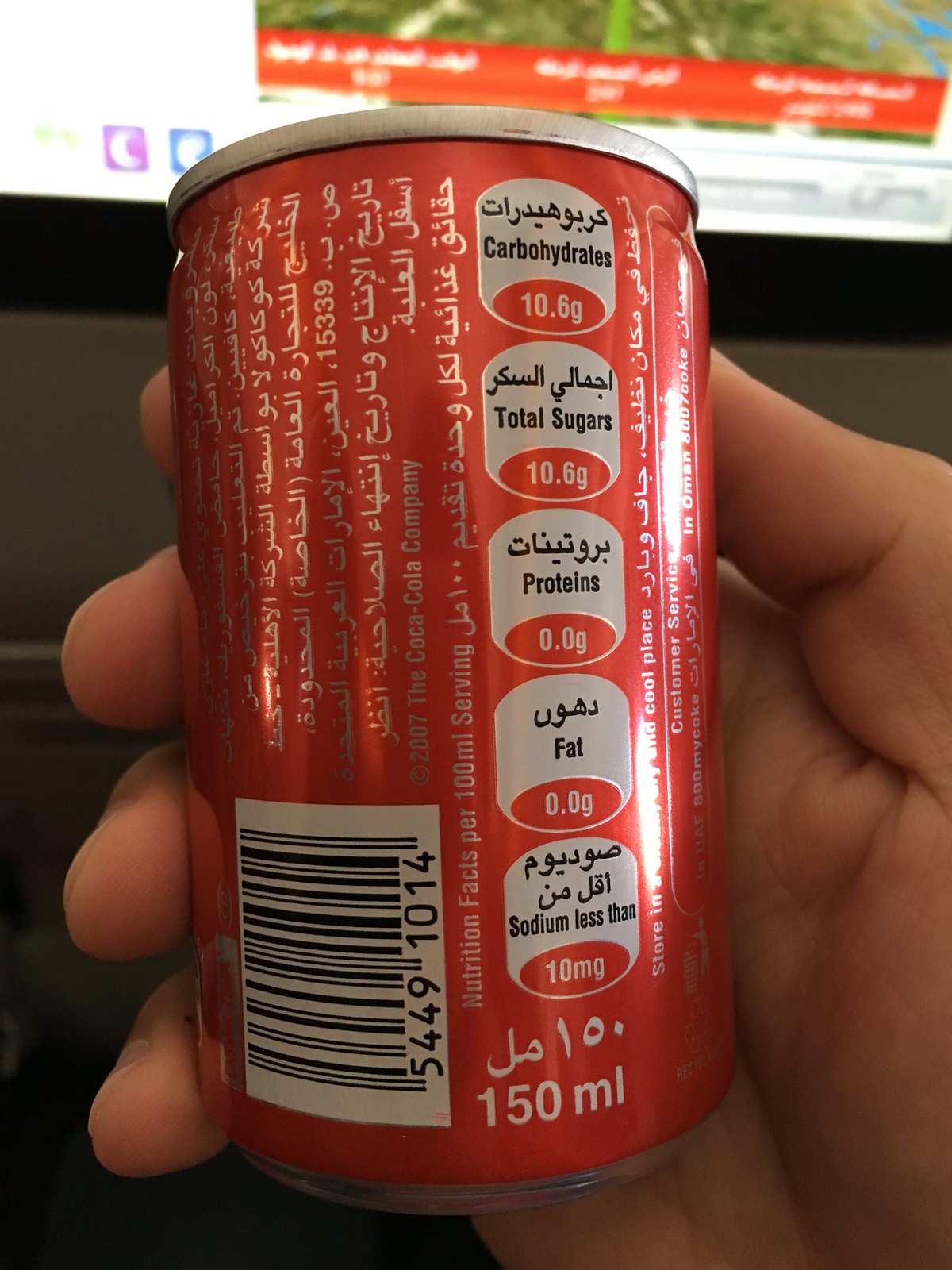The photograph prominently features a close-up of a right hand holding a 150ml red Coca-Cola can with a silver top and bottom. The can is predominantly labeled in Arabic, but includes some nutritional information in English, reading: carbohydrates 10.6g, total sugars 10.6g, protein 0.0g, fat 0.0g, and sodium less than 10mg. The can also has a vertically oriented barcode and a white UPC code. In the background, a computer screen is visible. The left hand likely holds the phone capturing the image. In the distant background, there appears to be a brown storefront with a white roof and a hint of a palm tree above. The can exhibits a detailed design with a recycling symbol and ingredients listed in Arabic, making it a cross-cultural product feature.